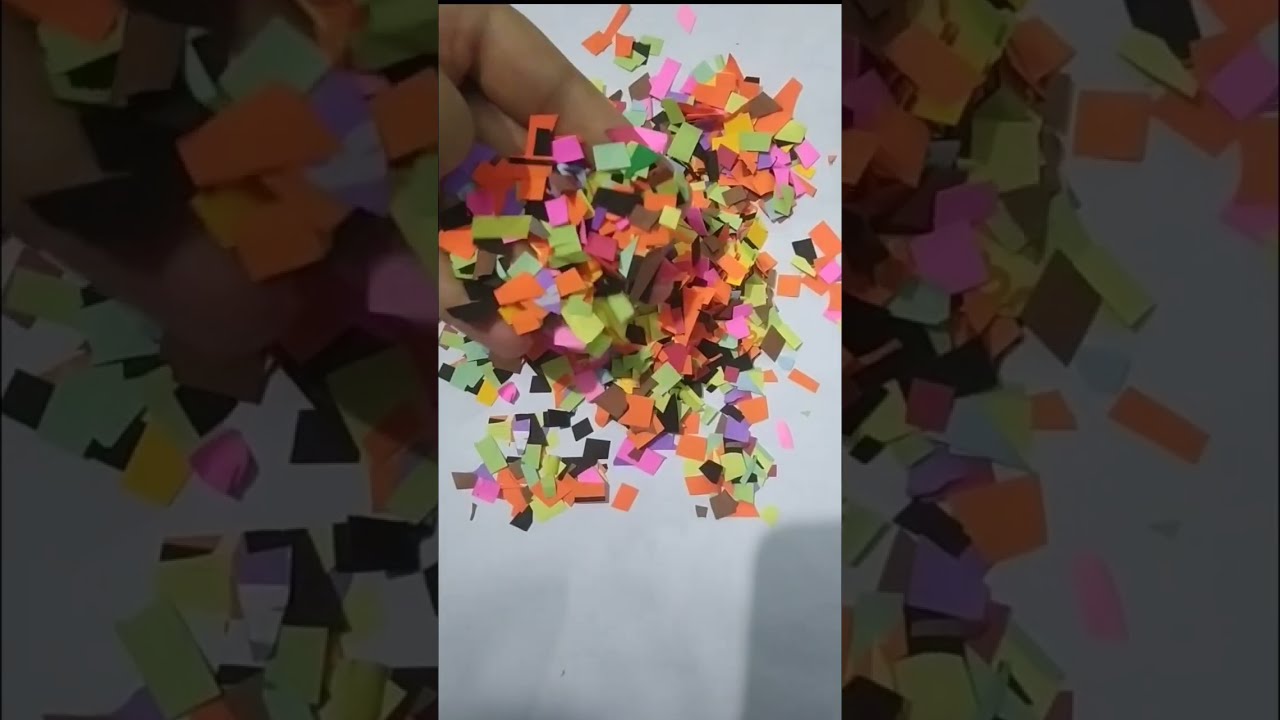In the center of this image, a left hand is holding an assortment of small, cut-up pieces of colorful construction paper, spread over a clean, white background. The pieces, reminiscent of confetti, come in a variety of shapes, primarily squares and rectangles, with a few triangles mixed in. The dominant colors include orange, purple, green, and yellow, alongside some black, pink, brown, and red. The hand, with fingers visible from the upper left corner, showcases the scale of these tiny fragments, highlighting their minuscule size. The left and right sides of the image feature darker, shaded rectangles with semi-transparent black filters, adding contrast to the vivid central display of the colorful cut-up paper. There is no text in the picture, which solely focuses on the vibrant array of confetti-like pieces in the hand against a stark white backdrop.